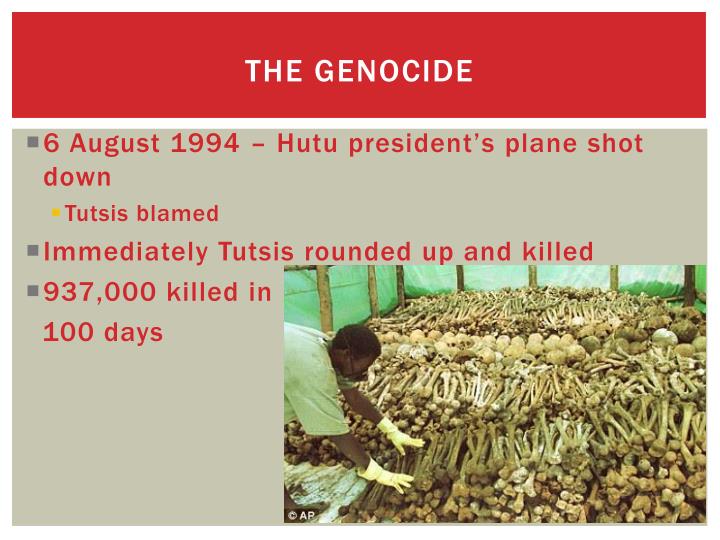The image is a poster, wider than it is tall, with a prominent banner at the top. This banner is a thick band of red, and in the center, it features white capital letters reading "THE GENOCIDE." A white line separates the banner from the rest of the poster.

Below the banner, the background shifts to light gray and is adorned with red text, structured into three bullet points. The first bullet point, introduced by a dark gray square bullet, states "6 August 1994 - Hutu's President Plane Shot Down." Below it, a bright yellow bullet point with the text "Tutsis Blamed" emphasizes the blamed group. The second dark gray bullet point follows, reading, "Immediately Tutsis Rounded Up and Killed." The final bullet point, also marked with a dark gray square, captures the staggering death toll: "937,000 Killed in 100 Days."

In the lower right quadrant of the poster, slightly extending above and to the left of the middle, is a disturbing photograph. It depicts a considerable pile of human bones, including skulls, all arranged neatly. A black man, wearing yellow gloves and a light green shirt, is seen leaning over the bones, touching them. Behind the pile of bones, there are fence posts and a light green fabric in the background, adding context to the somber scene.

The lower left quadrant of the poster remains mostly light gray, intersected by the text, especially the line "Immediately Tutsis Rounded Up and Killed," and the photograph occupying a significant portion of the bottom half. The gruesome yet meticulously organized image, combined with the harrowing statistics and events described, starkly captures the gravity of the genocide.